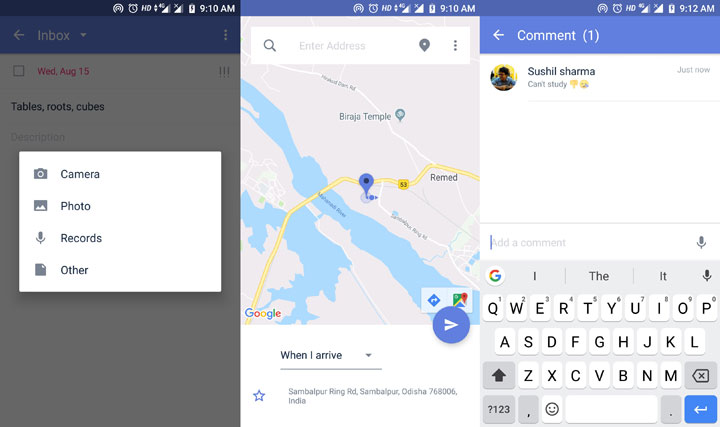The image consists of three screenshots from a mobile device, possibly a phone or a tablet, arranged side by side.

**Left Screenshot:**
- Background displaying an email inbox interface.
- Prominent header stating "Inbox."
- Date marker "Wednesday, August 15th" highlighted in red but not selected.
- Email subjects listed below, including one titled "Tables, Roots, Cubes."
- Foreground shows a white options box with selections for "Camera," "Photo," "Records," and "Other."

**Middle Screenshot:**
- Display of Google Maps.
- Key locations highlighted include "Biraya Temple" or "Biraha Temple" and "Remit."
- Above the navigation options, it mentions "When I arrive."
- Detailed route indicator pointing to "Zambulpur Ring Road, Odisha, India."

**Right Screenshot:**
- Open comment interface on a social platform or app.
- Username "Sushil Sharma" has posted "Can't study" followed by a sad face emoji and a thumbs down emoji.
- On-screen keyboard is visible, and the cursor is placed in the comment input box, ready for typing.

This detailed arrangement provides an insightful look into the various screen activities, showcasing a blend of email management, navigation, and social interaction.